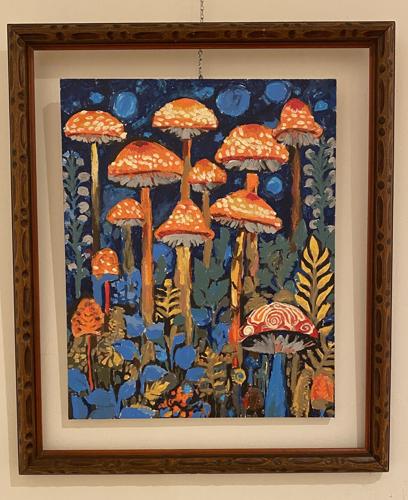The image depicts a photograph of a framed artwork in portrait orientation. The piece is enclosed in a wide, dark wooden frame with a cream-colored mat, accentuating the primary subject: an intricate painting of a mushroom-laden forest scene. The central focus of the artwork features numerous orange-capped mushrooms adorned with yellow dots, rising from various points within the composition. Interspersed among the mushrooms are stems in hues of brown, orange, and yellow. At the bottom, sky-blue flowers and a blue-stemmed mushroom emerge from the right corner, complemented by a golden yellow fern. Additionally, vibrant foliage in greens, blues, and reds embellishes the scene. The background is a dark blue, peppered with abstract lighter blue shapes and cream-colored flowers on stalks, framing the mushrooms. The painting showcases a blend of watercolor and oil-based techniques, emphasizing a photographic representational realism style. Notably, there is no text within the image, allowing the natural elements and rich details of the mushrooms and surrounding flora to captivate the viewer.